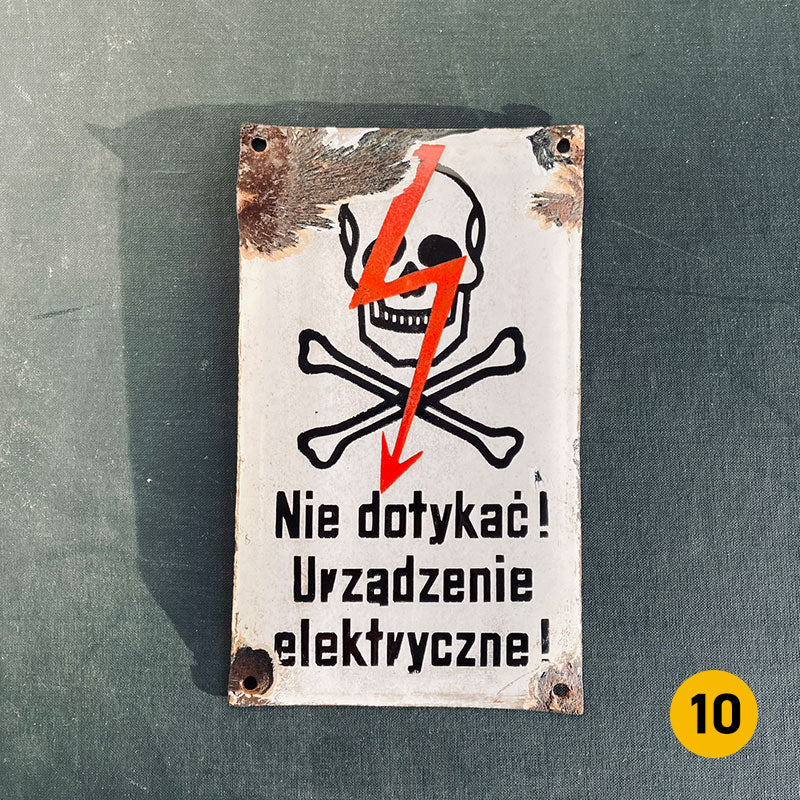This is an image of a white sign with peeling paint at the corners, mounted against a raggedy, possibly cloth background in a teal green color. The sign features a graphic of a skull and crossbones in black, with a prominent bright orange zigzag resembling a lightning bolt arrow pointing downwards towards some black text in a foreign language, possibly indicating a warning about an electric risk. The text includes an exclamation point. There are four holes, one in each corner of the sign, suggesting it was previously hung. In the lower right corner, the number "10" is displayed in black lettering within a burnt orange circle, which might indicate it is item number 10 in an exhibit or a catalog item. A shadow cast by the sign is visible due to the light shining on it.